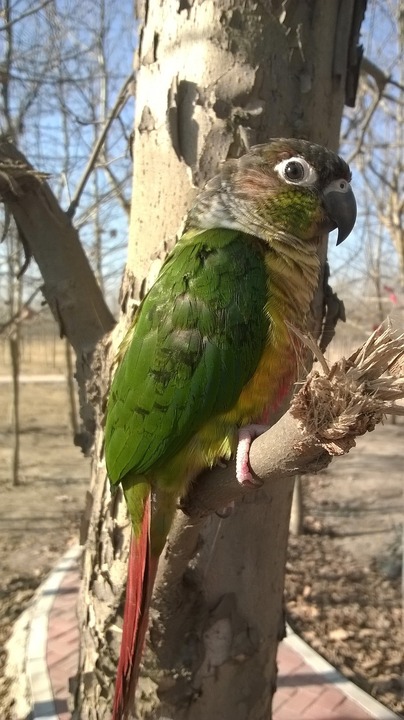This image depicts a medium-sized parrot perched on a broken limb of a tree, against a backdrop of a winter landscape. The parrot, positioned in profile, showcases its colorful plumage with striking green wings, a yellow-tinged chest, and a long, red-tipped tail feather. Its beak is curved and black, complementing its black eye that is encircled by a distinctive white ring. The bird grasps the branch firmly with its talon claws, and appears to have nibbled at the wood, adding to the branch's worn look. Surrounding the parrot is a scene with bare trees, a dirt ground, and a winding stone walkway. The muted tones of the image emphasize the season's stark beauty, while a clear blue sky offers contrast. The parrot's perch—the branch of a sickly-looking tree with peeling beige bark—adds texture to this serene, outdoor setting.